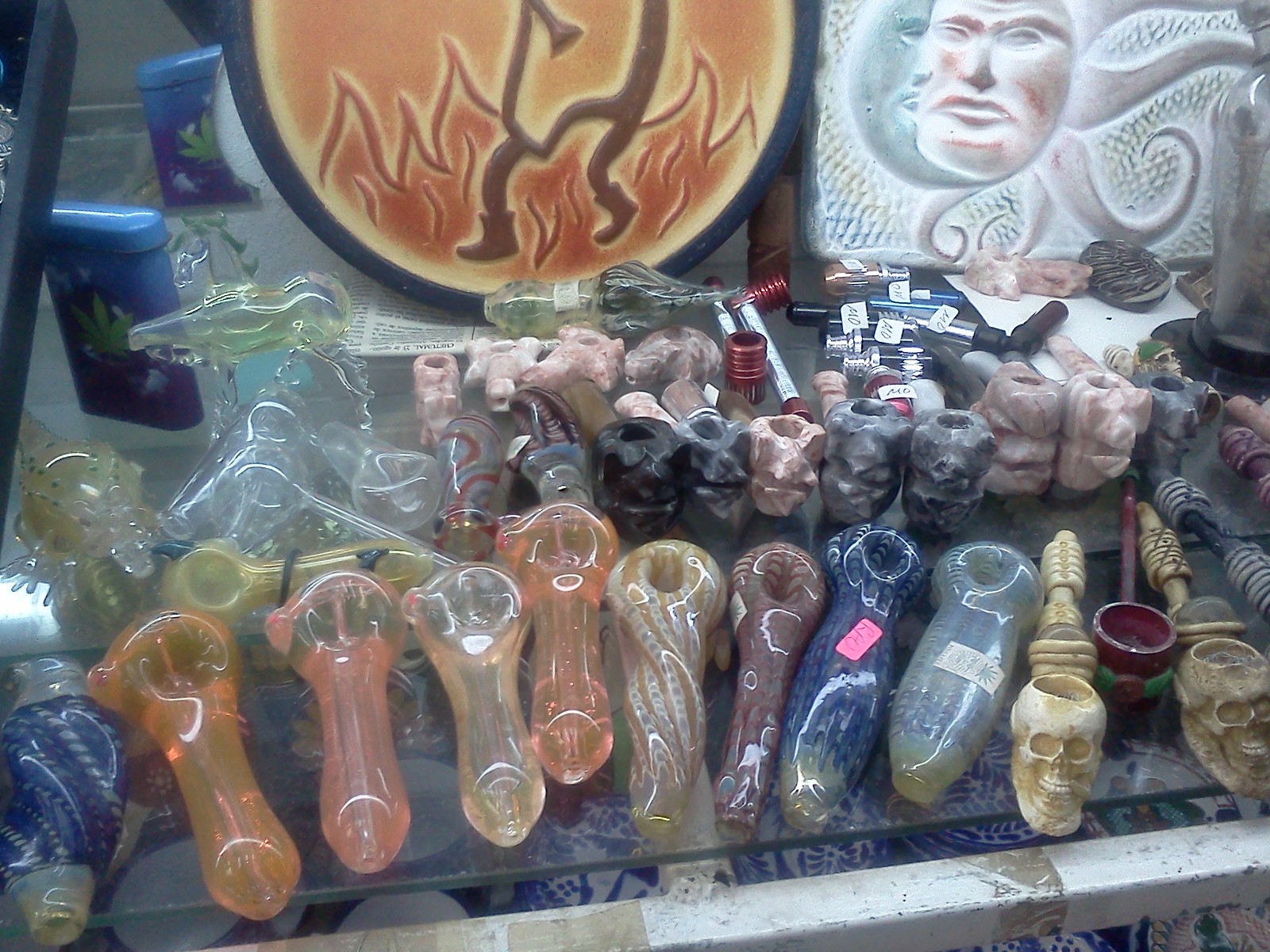The image depicts an eclectic-looking shop, likely specializing in smoking paraphernalia such as marijuana products and vaping accessories. On a glass display table, an assortment of hand-blown glass pipes are showcased, featuring vibrant colors like blue, pink, orange, cream, black, and red. These pipes vary in shape, some resembling donuts with a hole in the center, while others look like rods or spoons. Additionally, the display includes pipes adorned with skulls and some that appear to be made of stone. Beside the pipes, there are tins marked with marijuana leaf symbols, suggesting marijuana-related products. The table also holds various pottery-esque items and other intriguing objects, including a couple of striking artworks—one depicting feet engulfed in fire with dark orange to red hues, and another image with rays that might resemble a mosque painting. A large orange shield-like object with fire motifs and a peculiar mask-like face in the background adds to the store's diverse and intriguing ambiance.